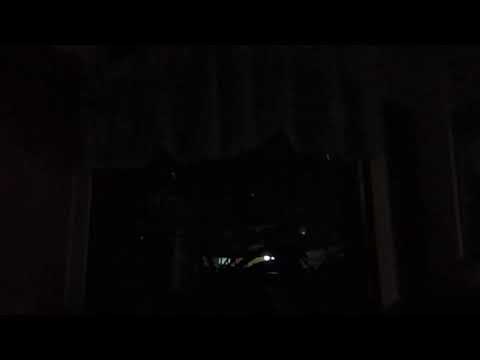This image is an exceptionally dark photograph, making it challenging to discern whether it is taken indoors or outdoors. The predominant color is black, but there are a few small areas that provide minimal illumination. Near the bottom center of the image is one bright light, accompanied by a few tiny white pinpoints resembling stars scattered in the darkness. Just off-center, there are white streaks, possibly light reflections. On the left and right edges, vague dark gray shapes hint at the presence of pillars, adding some faint structure to the scene. Most of the image remains obscured, with insufficient light to clearly reveal any details. There is also a suggestion of a white outline on the side and an indication of something that might read "HD," speculated to resemble a dimly lit car dashboard at night. Overall, the image is a dim, ambiguous depiction that leaves much to the imagination.